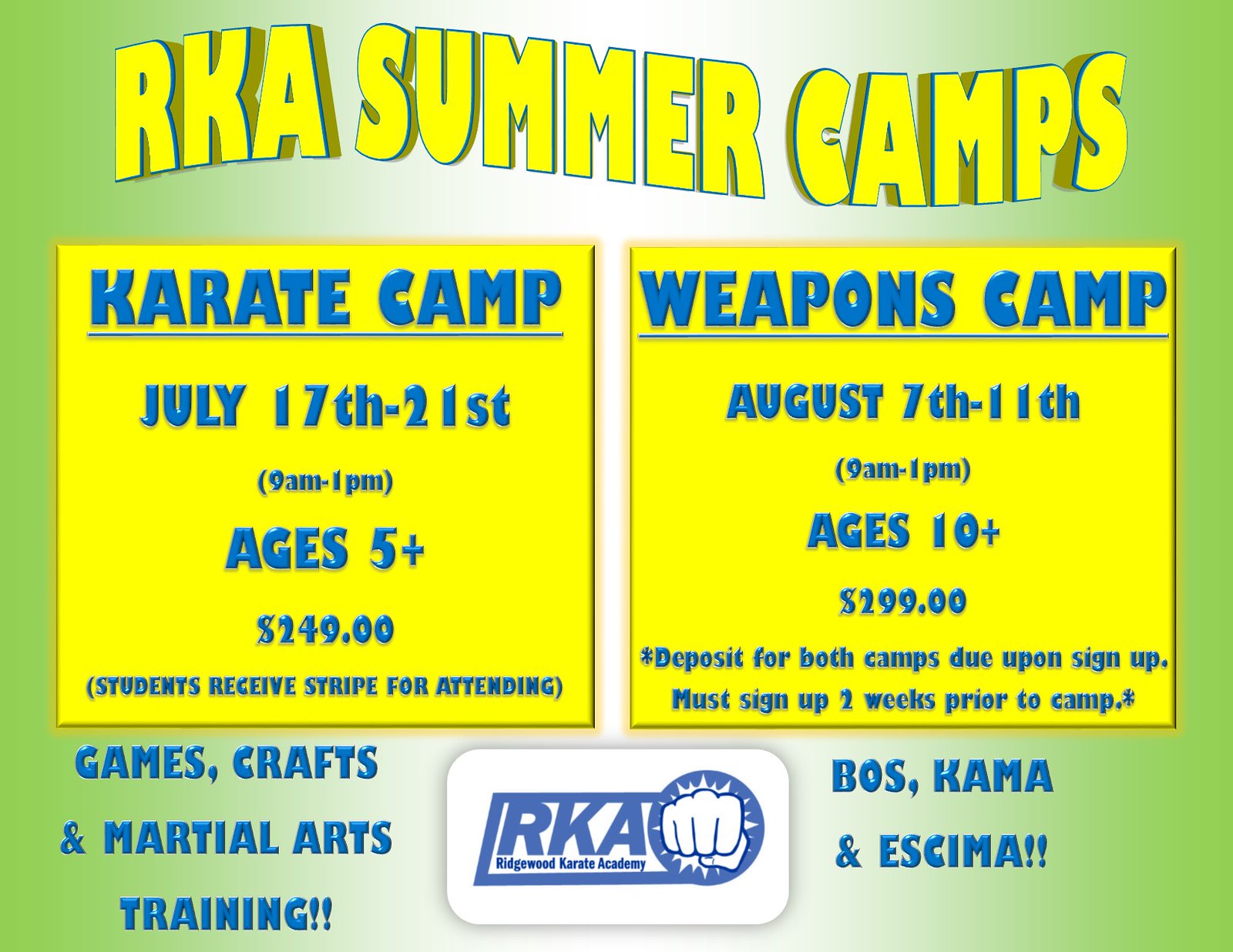The advertisement for RKA Summer Camps features a predominantly green background with a white stripe down the center, creating a green-white-green pattern. At the top, in yellow lettering, it reads "RKA Summer Camps." The middle section of the image is divided into two yellow-bordered squares. 

The left square, labeled "Karate Camp," lists the dates "July 17th to 21st" and the time "9 AM to 1 PM." It is open for ages 5 and up and costs $249. It also notes that students will receive a stripe for attending.

The right square, labeled "Weapons Camp," lists the dates "August 7th to 11th" and the time "9 AM to 1 PM." This camp is for ages 10 and up and costs $299. Important details include that a deposit for both camps is due upon sign-up and participants must sign up two weeks prior to camp. The camp will include games, crafts, and martial arts training.

At the bottom of the image, an icon of a sketch outline of a fist with explosion marks around it appears, symbolizing action and strength. Next to the fist, "RKA Ridgewood Karate Academy" is written. Additional affiliations, BOS, KAMA, and ESIMA, are also mentioned.